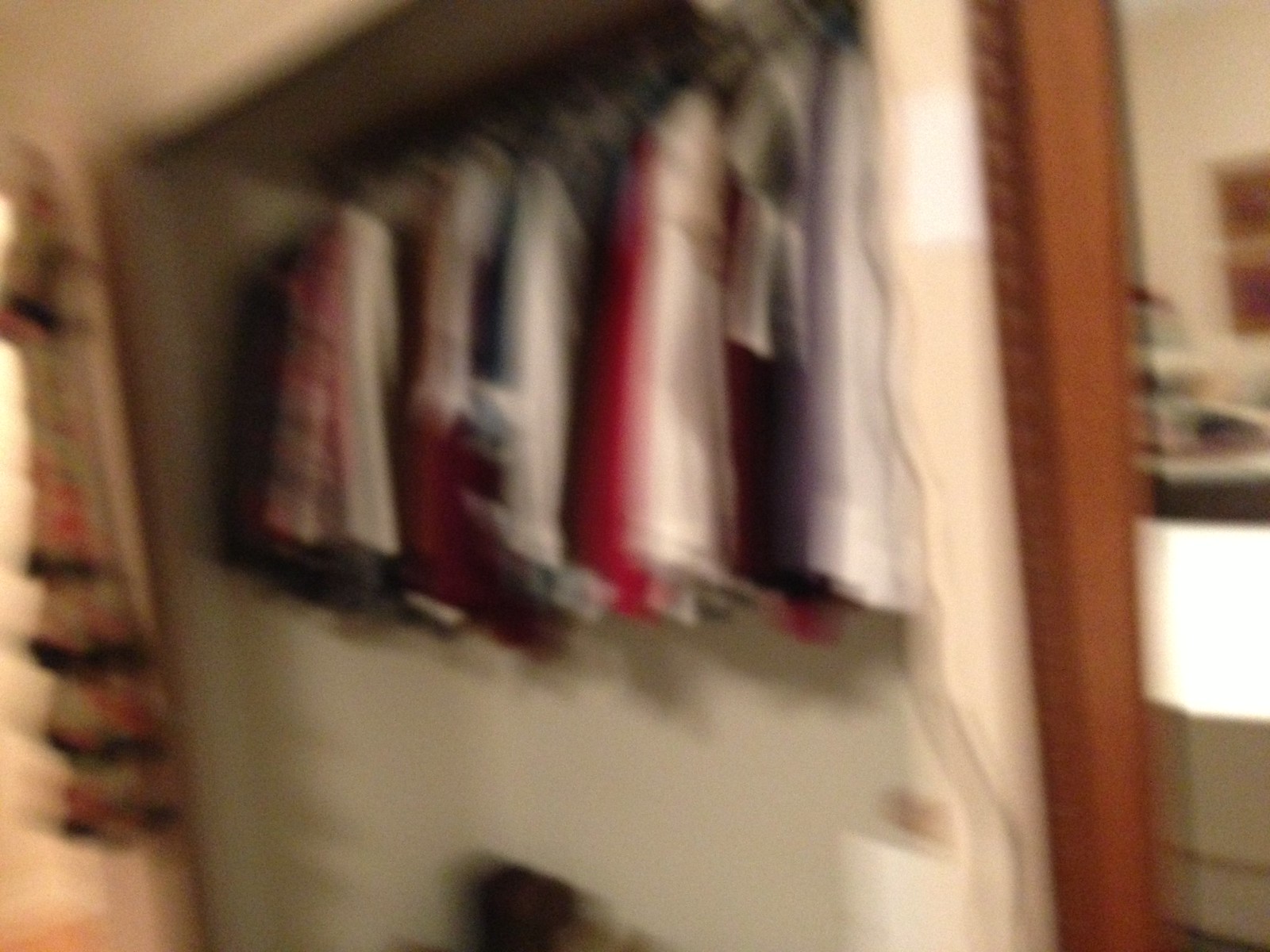This image depicts a dimly lit, blurry interior of someone's double-door closet, although the doors themselves are not visible. The closet is lined with an assortment of clothing, predominantly shirts, all meticulously hung on hangers near the top, close to the ceiling. Below the hanging clothes, there is a white object accompanied by an indistinguishable item. On the left side of the image, a portion of a curtain can be seen draping over a window, adding a touch of soft texture to the scene. On the right, a robust brown wooden door frame leads the eye towards a white item in the background. Above this, an opening is visible, possibly leading into another room or reflecting an adjacent space via a mirror on the wall.